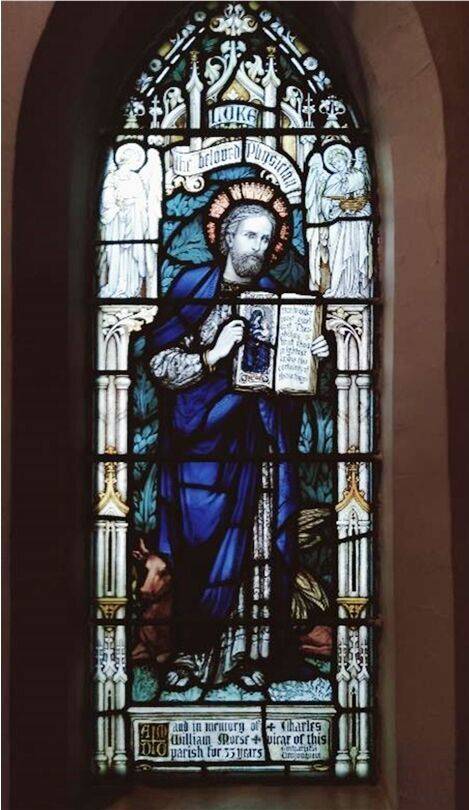This portrait-oriented photograph showcases a striking stained glass window set in a brown church wall, visible on either side of the image. The window, fashioned in a bullet shape, predominantly features hues of white with accents of green, blue, and gold. The central focus is a detailed depiction of a religious figure, likely Jesus Christ or possibly the gospel writer Luke, dressed in a blue robe. He stands holding an open book, revealing a picture on the left page and text on the right. A gold halo crowns his head, set against a light blue, feathery background. Below his feet, partly visible under his robe, are sandals. 

Surrounding the central figure, white-winged angels with black outlines appear to watch over him, adding to the window's intricate design. At the top, a banner reads "Our Beloved," though the subsequent text is indistinct. Similarly, an inscription at the bottom is rendered in black text that is too small to decipher. Through the convergence of artistry and spirituality, the window projects the visual essence of spreading the word of God, embodied in the form of this sacred and elaborate stained glass mural.